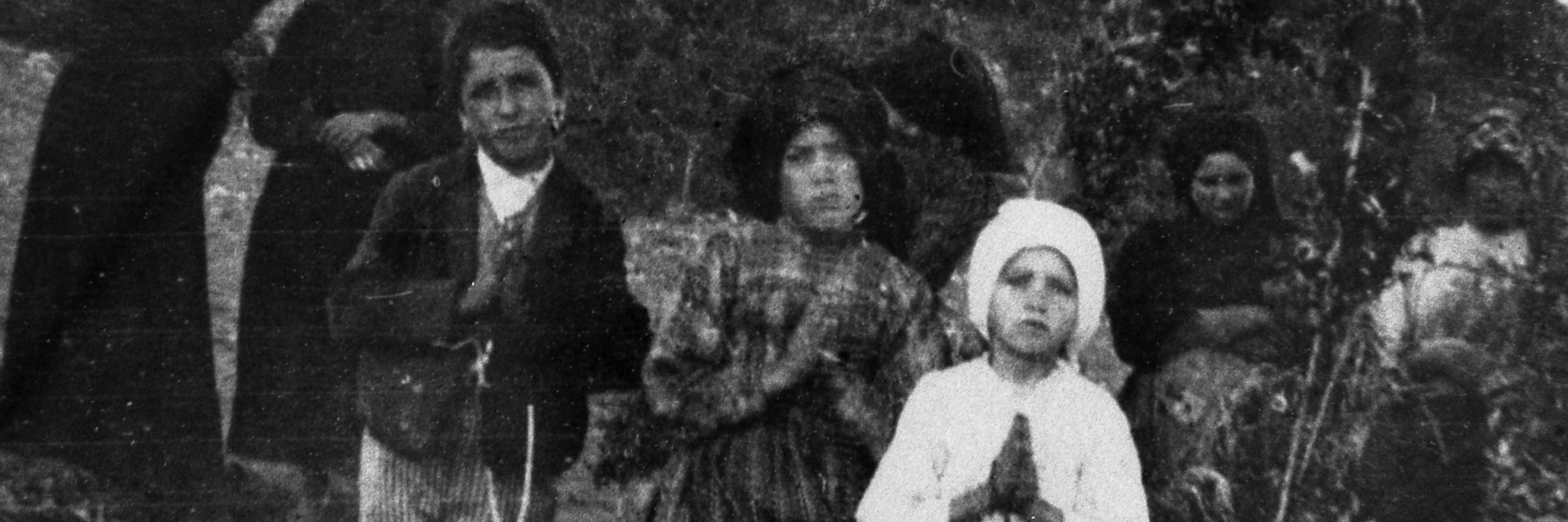In this grainy black and white image, which evokes memories of miraculous events like the Fatima apparitions, a poignant scene unfolds. Dominating the foreground is a young girl with a solemn expression, wearing a form-fitting white headscarf and a long-sleeved white dress. She appears to be praying, her hands clasped in front of her. 

Behind her, four figures stand in a row, their varying ages suggesting a mix of children and young teenagers. On the far left, a boy in a black jacket with a white collar and striped pants mirrors the prayerful pose. Next to him is a girl in a black headscarf and long-sleeved checkered shirt, also praying, her expression mirroring the somber mood. To her right, another girl is dressed in a black headscarf and a black outfit, while the far-right figure wears a checkered head covering and a white dress that may have a black skirt, though this part is slightly fuzzy.

The background reveals an outdoor setting with trees and bushes, reinforcing the natural, serene atmosphere. In the upper left corner, two more figures, their legs extending the height of the picture, wear dark attire, further adding to the contemplative mood of the scene.